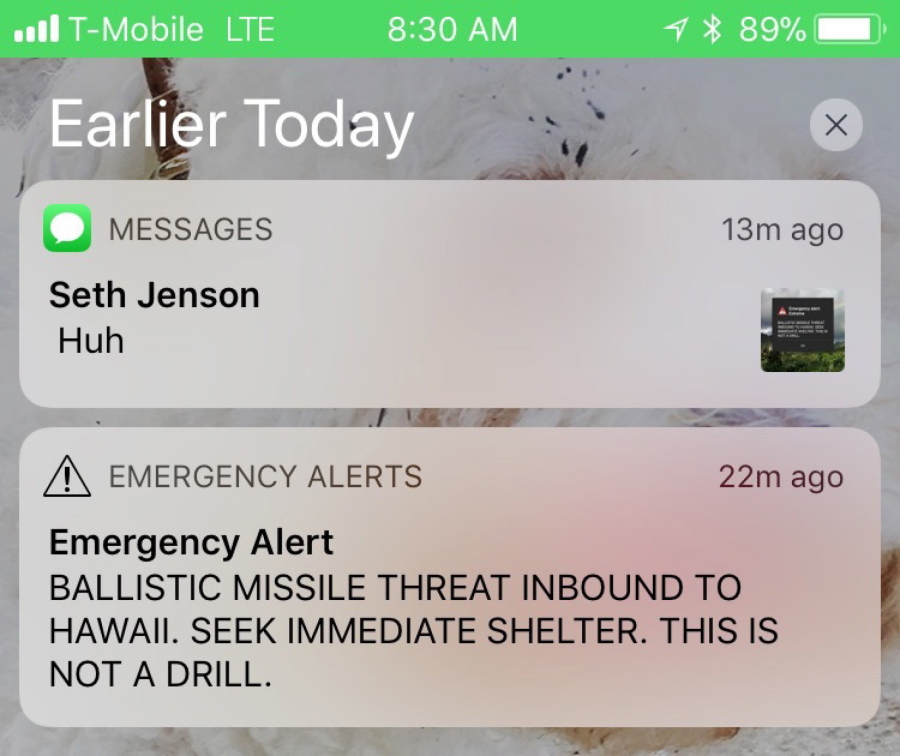The image is a detailed screenshot of an iPhone screen with several distinct elements visible. At the top-left corner, it displays "T-Mobile LTE," with the time as "8:30 AM" and the battery level at 89%. The notifications area shows messages and alerts from today. A message from Seth Jensen, sent 13 minutes ago, simply says "huh" and includes a small, indistinguishable picture that appears to be a billboard. Below this message, there's a stern emergency alert sent 22 minutes ago, which reads, "EMERGENCY ALERT: BALLISTIC MISSILE THREAT INBOUND TO HAWAII. SEEK IMMEDIATE SHELTER. THIS IS NOT A DRILL," all in capital letters for emphasis. The top bar also features icons for GPS and Bluetooth. The background wallpaper partially visible behind these notifications is white with an artistic design.